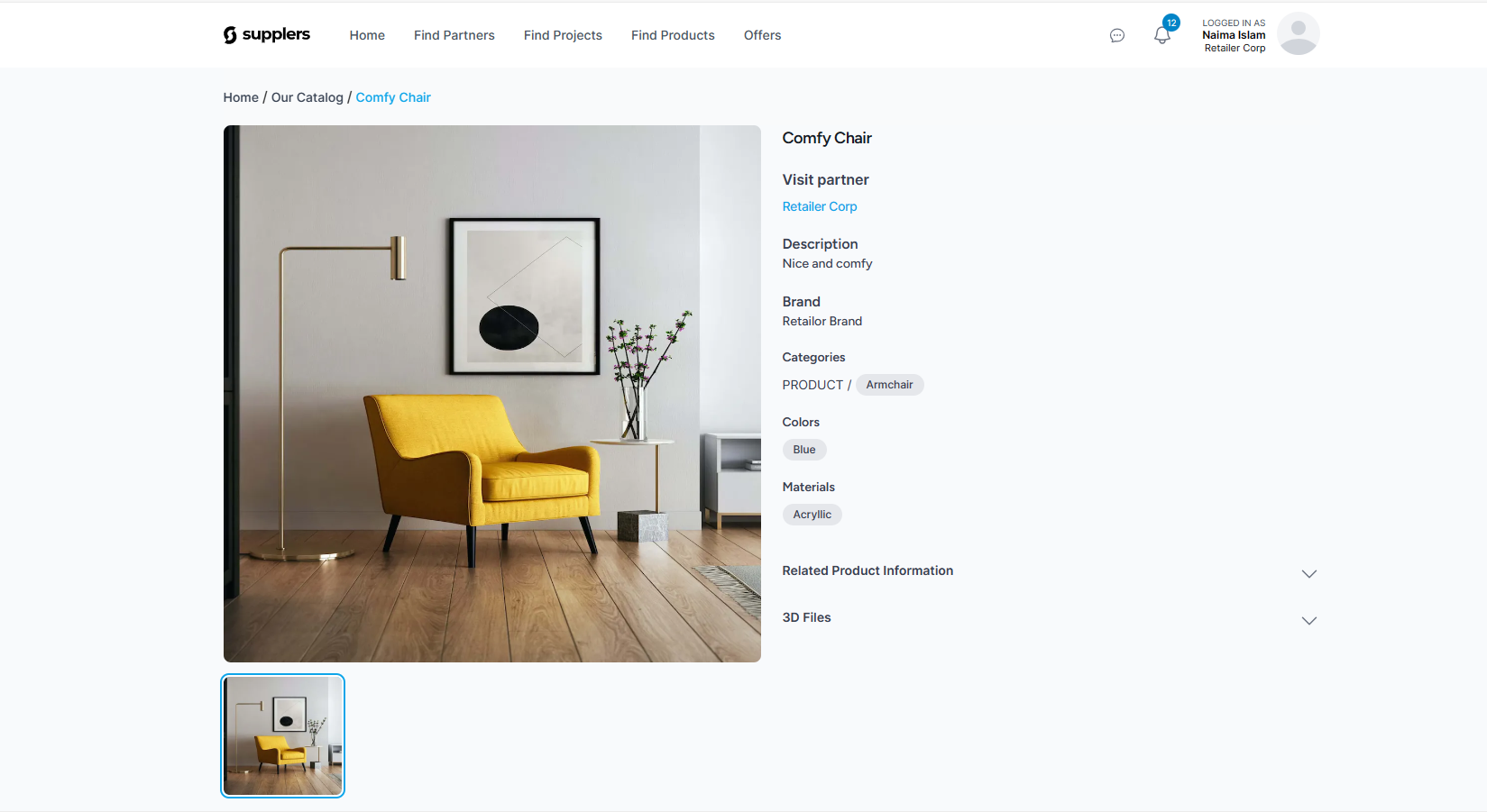The image showcases the homepage of a website named "Supplers," prominently displayed in black font at the top left corner. To the right of the site name, a navigation menu includes tabs with categories: "Home" in gray, "Find Partners," "Find Projects," "Find Products," and "Offers." The top right-hand side of the page indicates that the user Neema Islam is currently logged in.

The main content features a photograph of a living room area. The room includes a yellow armchair next to a gold lamp. A black-framed print adorns the white-painted wall, and a side table beside the chair holds a vase with flowers. The area features light brown wooden floors accompanied by a rug.

Adjacent to the photograph, the text reads "Comfy Chair," followed by "Visit Partner." Below this, in blue, it states "Retailer Corp," and further down in black, it provides a description: "Nice and Comfy." The brand "Retailer Brand" is mentioned, categorized under "Product Armchair" with the color listed as "blue acrylic." Additional information includes related product details and availability of 3D files.

Above the photograph, a breadcrumb trail in blue and black indicates the page's navigation path: "Home / Our Catalog / Comfy Chair."